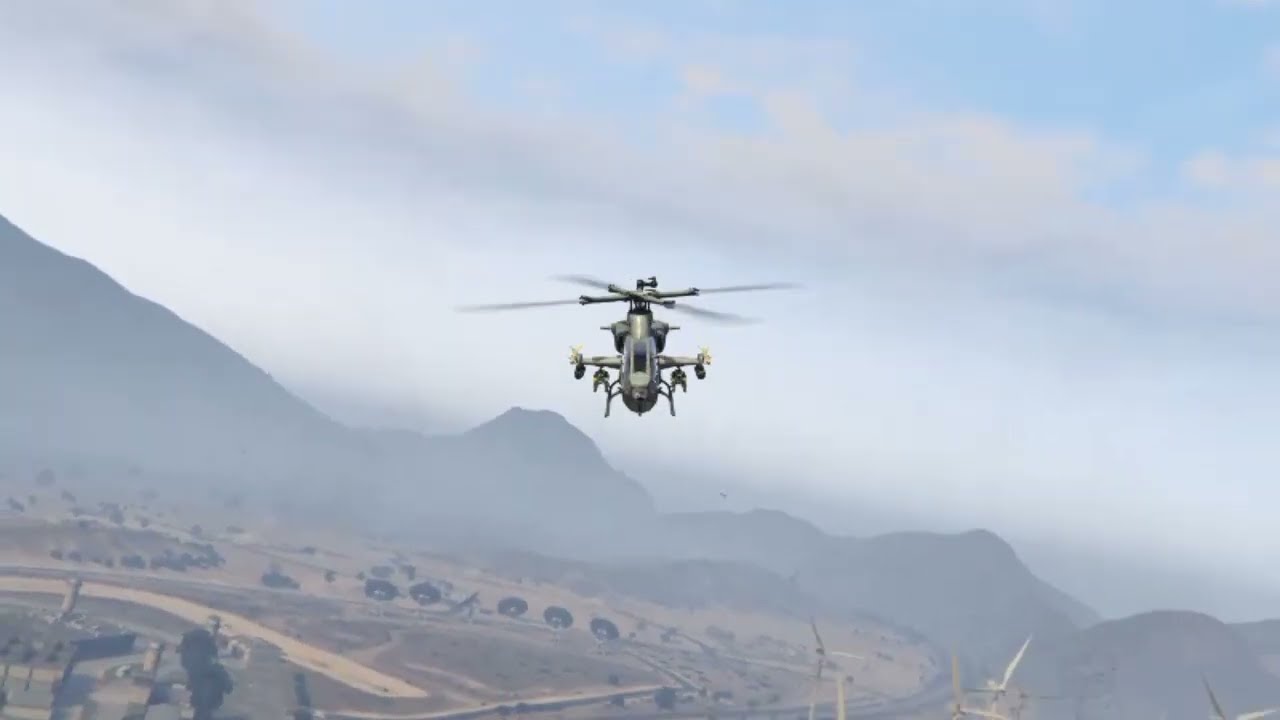This detailed screenshot from a video game showcases a light grey helicopter centered in the frame, flying directly towards the viewer. Its spinning rotors appear blurred, indicating motion. The helicopter is equipped with two turrets on either side. Beneath it, the ground area is a mix of empty desert terrain with sparse buildings, including a watchtower in the bottom left corner and wind turbines in the bottom right. Further back, the landscape transitions to indistinct brown and dark green hues, dominated by mountain outlines shrouded in hazy visibility. Above, the sky is a mix of blue and white, with some clouds and a faint dusty fog.